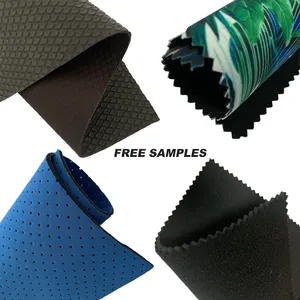The image features a small, square photograph with a white background, centered with the text "FREE SAMPLES" in bold black lettering. Surrounding this text in each corner are four fabric samples, each distinct in color and texture. 

In the top left corner, a ribbon-like, reversible fabric twists in an S-shape, exhibiting an olive green diamond pattern on one side and a burgundy or brownish color underneath. The sample in the top right corner is a tightly rolled fabric, showcasing black on one side and a plant-like design with various streaks of black, white, blue, and green on the other. The bottom left sample is also rolled and made of bright blue material, resembling foam with evenly spaced perforations throughout. Lastly, the bottom right fabric is black with rigid, jagged edges akin to a rubber mat or foam rubber, possibly folded for display. Overall, these samples seem to highlight a variety of textiles, potentially from a mill or store.